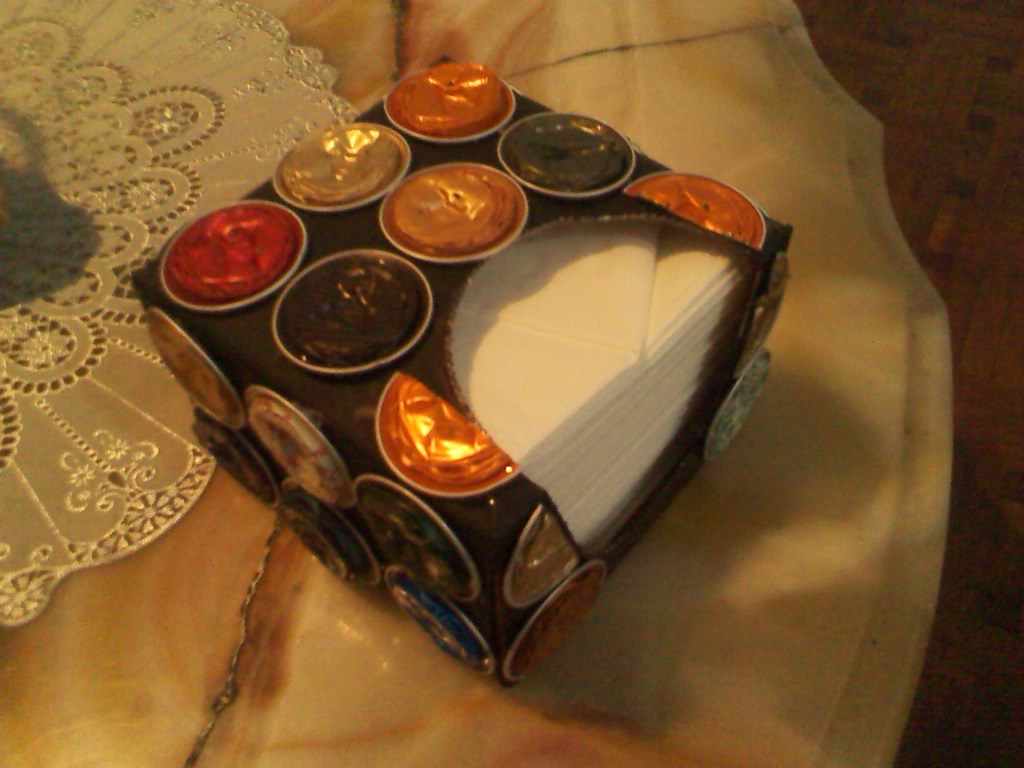This photograph, possibly captured with an older digital camera, showcases a grainy texture characteristic of aging digital images, with noticeable multi-colored film grain. The image, tinted in a reddish sepia hue likely due to artificial lighting, centers on a distinctive decorative tissue box. The tissue box, painted black, is a cardboard cube adorned with reflective circular ornaments that resemble metal caps in shades of red, orange, yellow, and brown, giving it a mosaic-like appearance. The white tissues within the box protrude from a central opening.

The tissue box is positioned prominently on a table, which appears to be made of a beige and brown ceramic or marble-like material with uneven, swirling patterns and a notably irregular edge. This unique table, possibly repaired or cracked, adds to the eclectic feel of the scene. On the table, towards the top left of the image, lies a lacy doily, further contributing to the photograph's ornate detail.

In the background on the upper right edge of the snapshot, the dark brown wooden flooring is partially visible, providing a contrasting backdrop to the vibrant and texturally rich elements in the foreground.